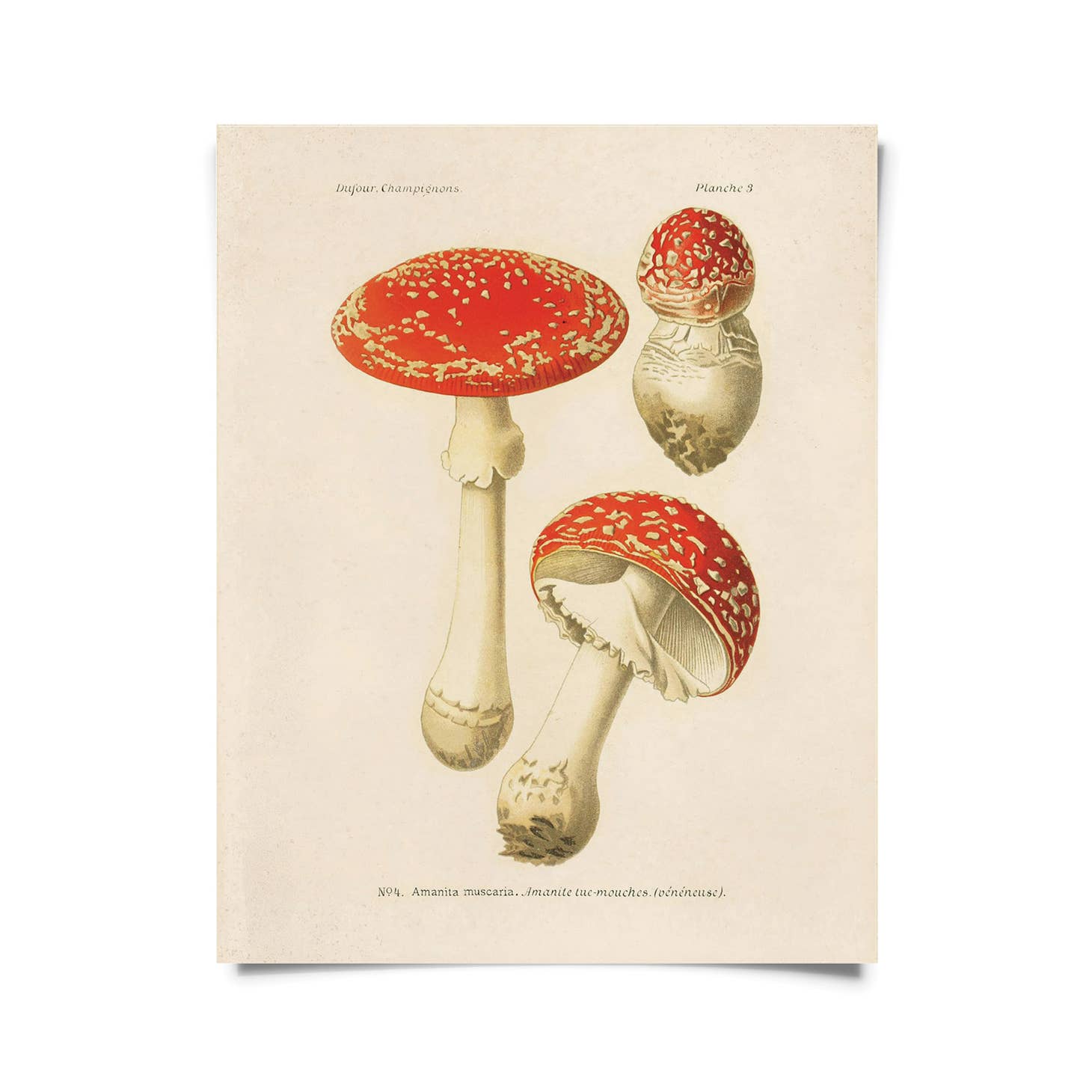The image depicts a detailed illustration from an old book or magazine, featuring three Amanita muscaria mushrooms at various stages of growth. The off-white, beige-colored paper sits against a white background, casting a soft drop shadow. In the upper left corner, text reads "défaut champignon," while the upper right corner says "Planche III." At the bottom, small lettering indicates "Number 4 Amanita muscaria."

The three mushrooms are skillfully illustrated in textbook style, each showcasing a different developmental phase. On the upper right is a young, tightly closed, egg-shaped mushroom with a bulbous base. The lower right depicts a medium-sized mushroom, its red cap speckled with white dots, dome-shaped, and the stem elongating. On the left side is a fully mature mushroom, with a broad, umbrella-like red cap covered in white specks, and a long, cream-colored stem that widens towards the base. This collection of meticulously detailed illustrations highlights the beauty and intricacy of Amanita muscaria mushrooms.